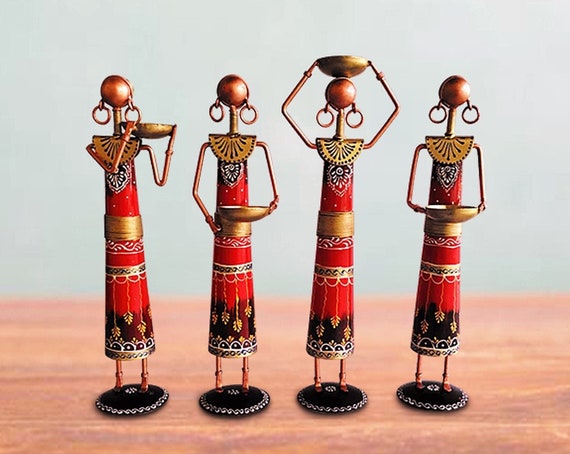The image depicts four stylized human figures resembling decorations possibly inspired by African, particularly Maasai, cultural attire. Each figure stands on a round black base and is likely crafted from wood, as suggested by their conical-shaped bodies and thin limbs. They are clad in matching red dresses with black patterns, adorned with golden hoop earrings, and collars resembling half-fan shapes, enhancing their regal look. These figures are faceless, with smooth copper or gold spheres for heads, and could be interpreted as carrying traditional items in a ceremonial manner. Each one holds a golden bowl differently: one lifts it to its neck, another cradles it at waist level, a third balances it on its head, and the fourth holds it in front with both hands. The scene is set on a wooden table against a gray background.